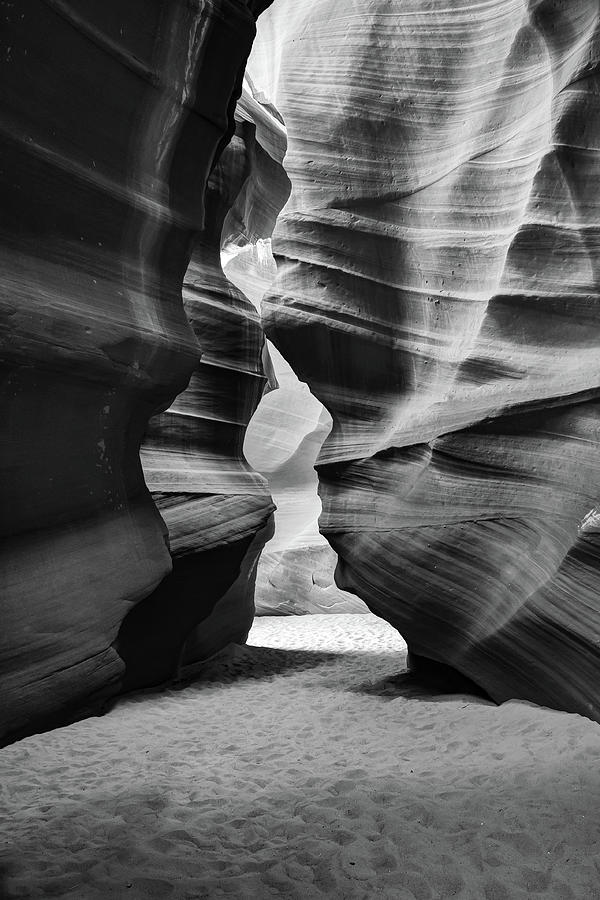This detailed black-and-white photograph captures the inside of a windswept cave that appears to be partially illuminated by natural light. The cave is constructed from smooth, slate-like rock walls that feature discernible horizontal ridges and varying layers, adding texture and depth to the scene. The cave floor is composed of fine sand, marked by numerous divot holes suggesting recent animal activity rather than human footprints. Light filters in from an opening in the center of the cave, creating a dramatic contrast between the darker left side and the more brightly lit right side of the rocks. The rectangular photo, taller than it is wide, guides the eye inward toward this tantalizing glimpse of brightness and additional sandy ground beyond the opening, evoking a sense of mystery and intrigue akin to scenes from caves in the American West.